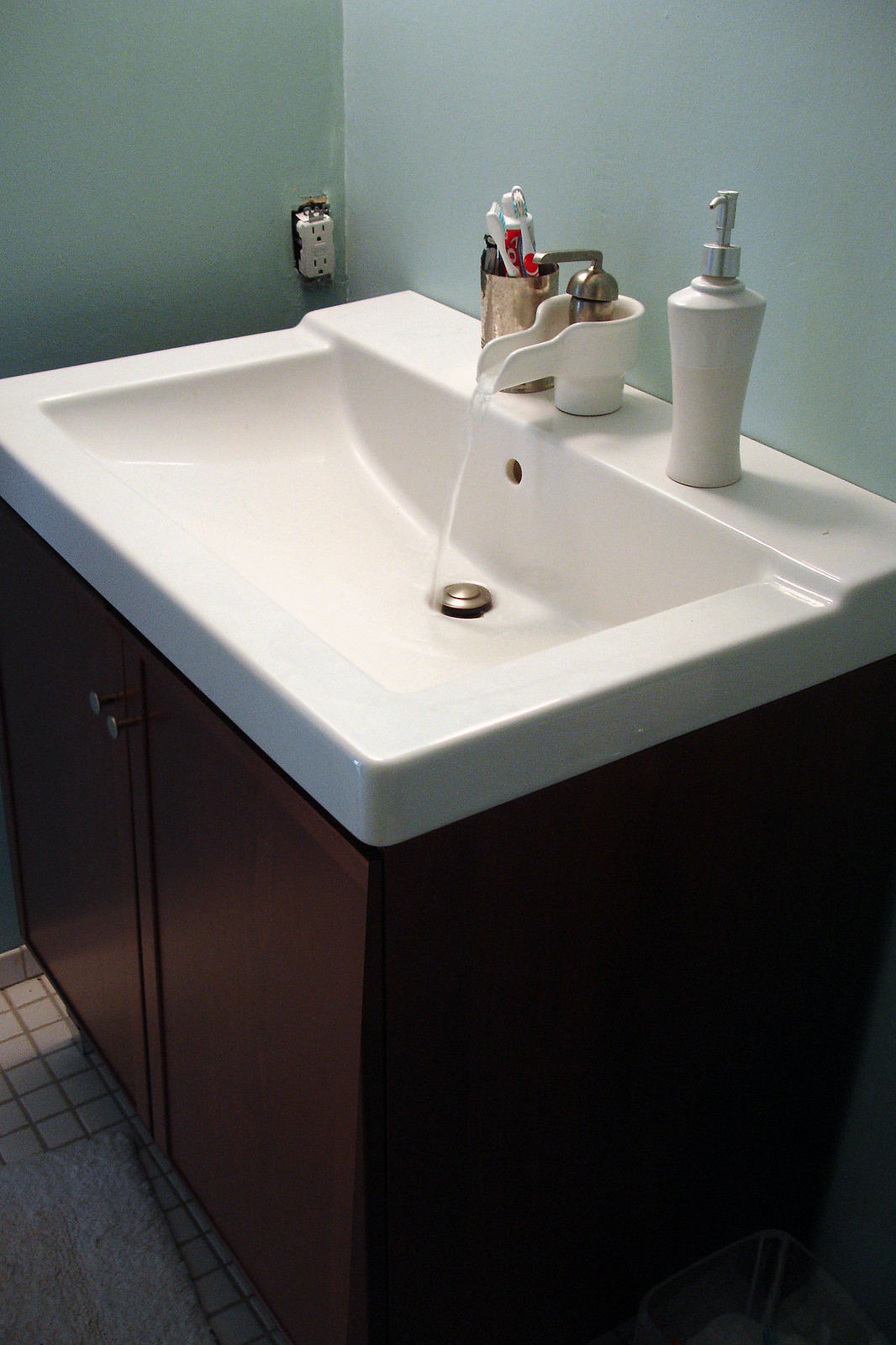This portrait-style photograph captures a close-up view of a bathroom sink with meticulous detail. The sink, made of white ceramic, is mounted onto a cherry wood cabinet. The backdrop is a soothing minty green wall, adding a fresh ambiance to the setting. Water is actively flowing from a white ceramic spout into the sink, creating a sense of movement. Adjacent to the spout sits a matching white ceramic soap dispenser, while a bronze cup filled with toothbrushes and toothpaste adds a touch of rustic charm. On the far end of the sink, a white electrical outlet is visible, while the cream-colored tile flooring completes the serene bathroom scene.